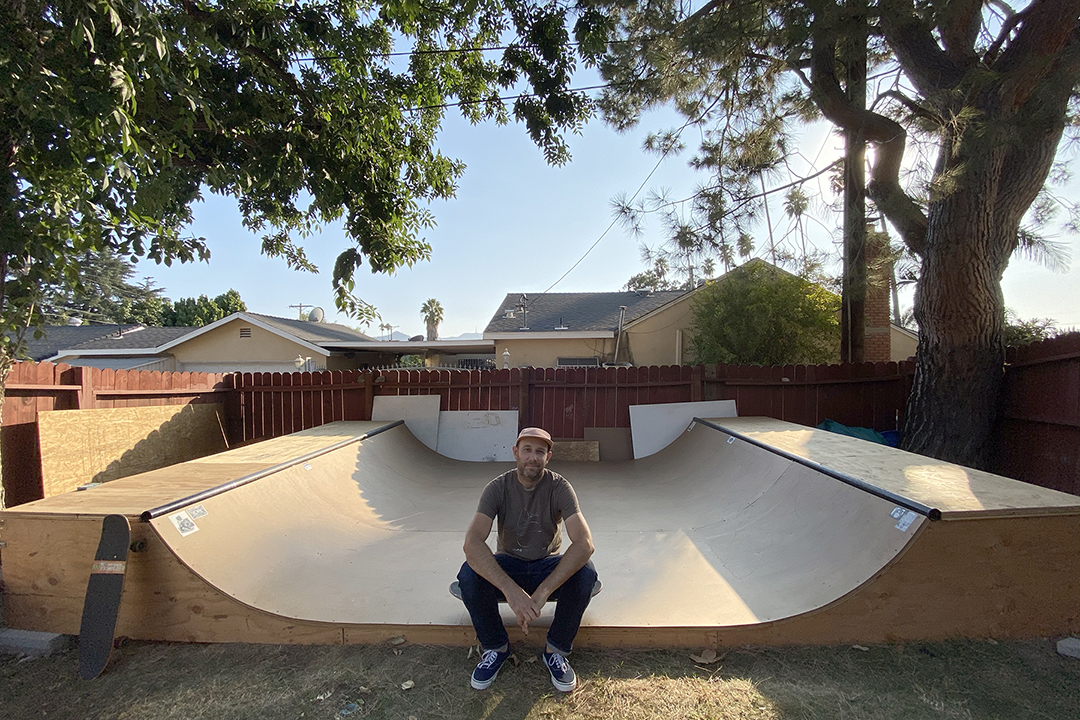The photograph depicts a detailed outdoor scene on a sunny day. The top half showcases a clear blue sky with some trees flanking the edges, partially outlining rooftops of nearby houses. Below this, a large, reddish-brown stained wooden fence stretches horizontally. Positioned in front of the fence is a wooden skateboard ramp, featuring a central dip that ascends on both sides.

At the center, a young man, who appears to be Caucasian and casually dressed, sits comfortably on the ramp. Donning a light reddish-toned ball cap, a light gray short-sleeved t-shirt, and dark blue jeans, he has a gentle smile with his head slightly tilted. His five o'clock shadow, peppered with gray, adds to his relaxed demeanor. Notably, his unusually large forearms and hands, possibly edited for effect, rest on his legs while his elbows are propped up. To the left side of the ramp, a skateboard leans against it.

The setting suggests a homemade ramp in a residential backyard; indicative elements include the grassy area under the man’s feet, the surrounding fencing, and the presence of trees and power lines in the background. The photograph combines elements of suburban tranquility with a hint of skateboarding culture.